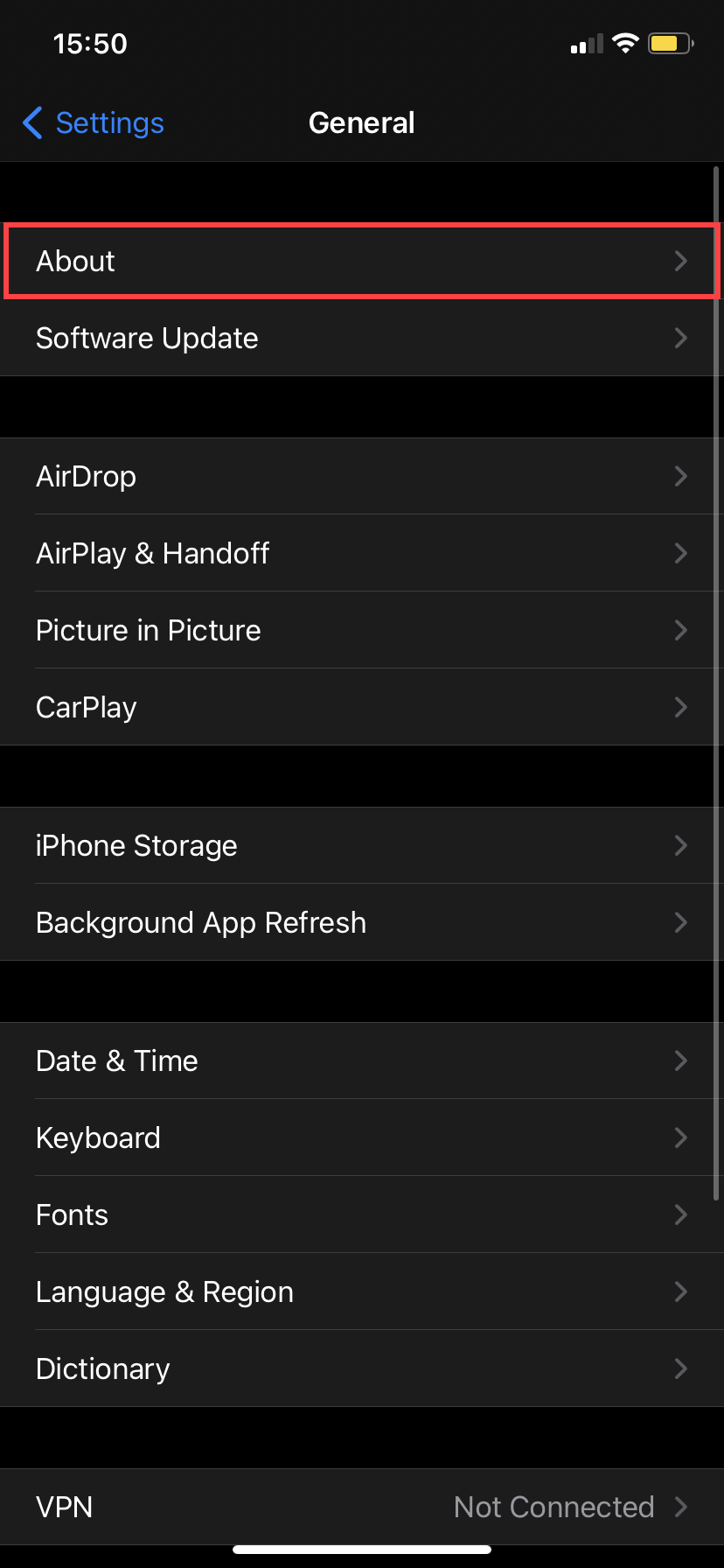The image displays a screenshot from a cell phone set against a solid black background. In the upper left corner, the time reads "15:50" in white text. The upper right corner features several status icons: two out of four bars for cell reception, an active Wi-Fi symbol, and a nearly full battery displayed through a battery icon.

Beneath these status indicators, blue text on the left reads "Settings" with an arrow pointing left, and "General" is centered below it. Directly under "General," a red border outlines the word "About" in white text.

A vertical list descends from "About" listing various menu items in white text:
- Software Update
- AirDrop
- AirPlay & Handoff
- Picture in Picture
- CarPlay

A thin black line separates these options from the next set of menu items:
- iPhone Storage
- Background App Refresh
- Date & Time
- Keyboard
- Fonts
- Language & Region
- Dictionary

In the lower corners, the screen indicates "Not Connected" in the lower right and "VPN" in the lower left.